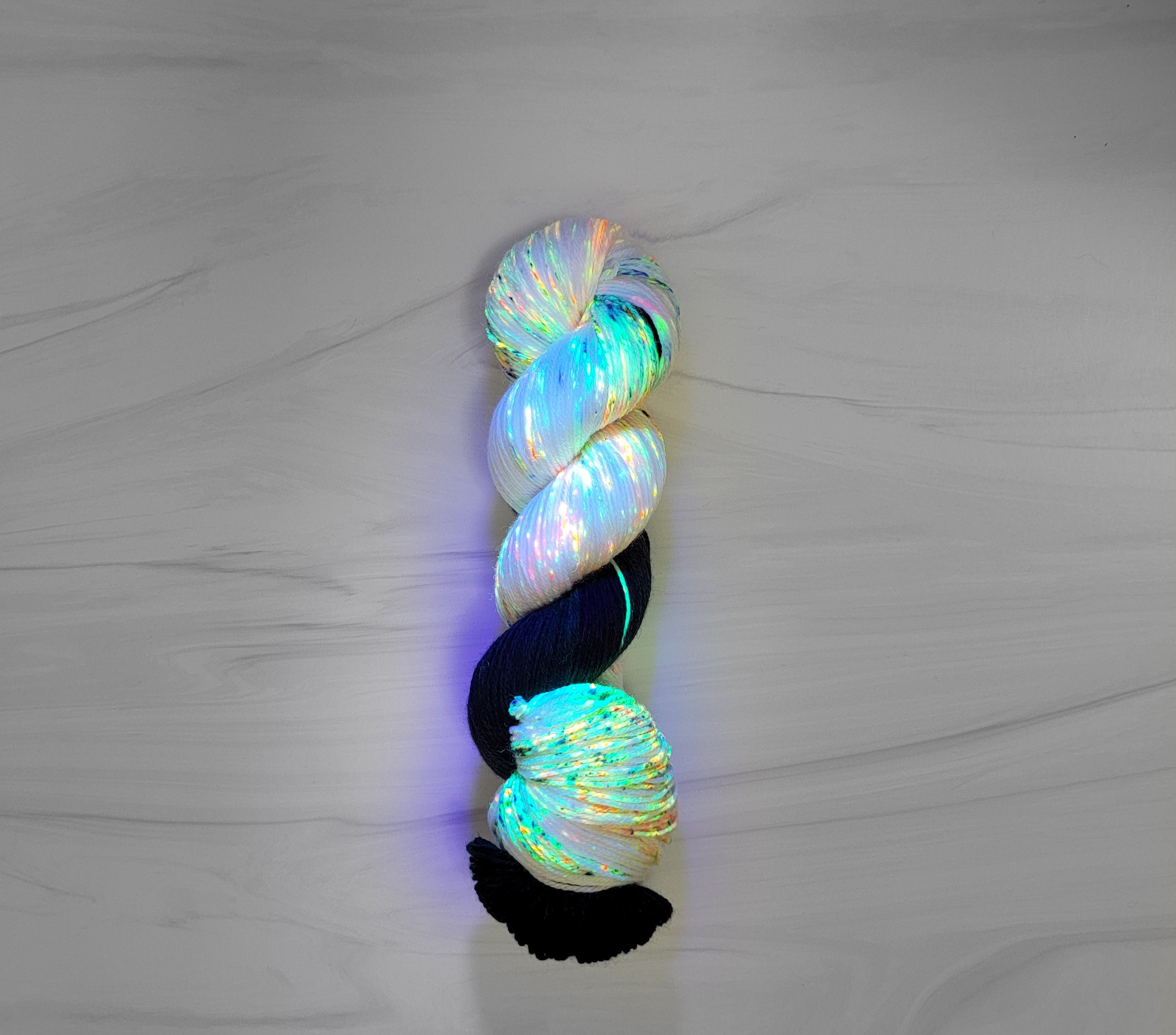The image is a square photograph of a sculptural art piece made from twisted yarn. The yarn is a combination of white, black, and various luminous colors including yellows, greens, light blues, aqua, and lavenders, giving it a glowing, almost metallic appearance. The illuminated effect suggests there may be lights integrated within the yarn. Placed at the center of the photograph, the yarn forms a rope-like structure that stands out against its background. The yarn is arranged on a flat surface that resembles white marble or light tan wood with a marble-like grain pattern. There is a distinct blue light shining onto the yarn, enhancing its vibrant hues and casting a subtle blue outline around it. The composition is minimalistic, placing full focus on the yarn with no other objects on either side, emphasizing its intricate and colorful details.